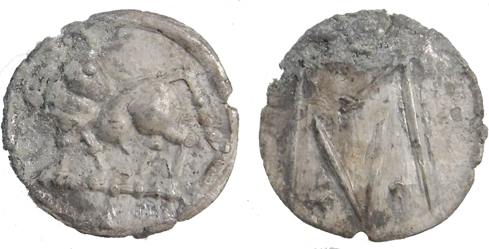The image depicts two ancient, corroded circular coins from an ancient culture, displayed on a white background. The coins are imperfect circles, each bearing cracks and notches along their edges, giving them a bronzed, worn appearance. The coin on the left is particularly challenging to interpret due to corrosion, but it appears to feature an indented design that might depict a person alongside an animal. This detail is elusive and open to interpretation, as the image is quite degraded. The right coin, presumably the back side, is rough with numerous lines and indentations, potentially representing sticks, swords, or abstract markings. The coins exhibit a dirty, brownish-gray color, and the suggestion of being stamped or carved adds to their mysterious and ancient allure.